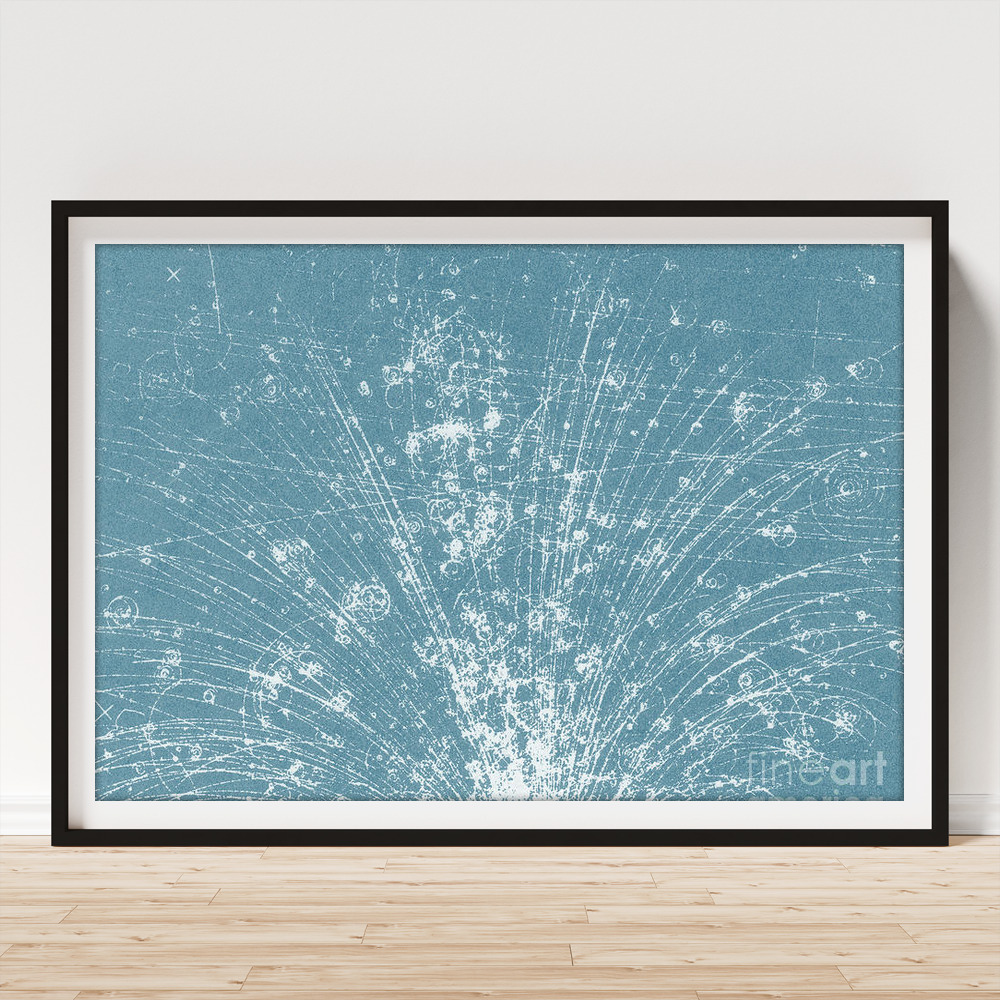This photograph captures an abstract painting resting on a very light, pine-colored hardwood floor, possibly part of a desk or the floor itself. The painting, framed with a black outer border and an inner white matt board, features a predominantly light slate blue background. The composition includes numerous vertical lines extending from a single apex point, resembling the way thin, bladed leaves of a plant fan out from the center. Interspersed among these lines are coiled, concentric circle shapes that swirl inward toward the center. Additionally, scratchy, random lines and varied straight and curvy lines, some resembling the shape of wheat fronds, are scattered throughout the image. The painting's lower right corner is marked with the words "Fine Art" as a watermark, and it is set against a clean white wall, emphasizing its intricate details and abstract nature.